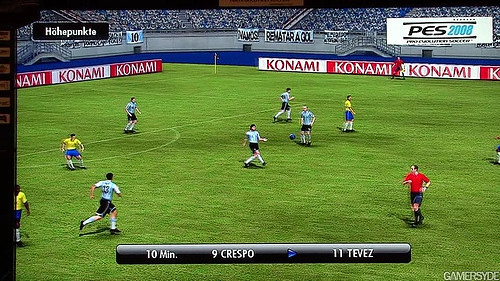This screenshot captures a moment from the soccer video game Pro Evolution Soccer 2008, produced by Konami. Despite being dated, the graphics manage to avoid a blocky appearance and feature characters with a moderate level of realism. The vibrant green soccer field is the backdrop for players in blue and white striped uniforms reminiscent of Argentina's national team, while opponents in yellow and blue outfits evoke Brazil's colors. Along the field’s perimeter, red and white Konami banners catch the eye, reinforcing the game developer’s presence. In the bottom right corner, a watermark from GamerSide is visible, marking the source of the screenshot. Additionally, a black bar at the bottom displays the in-game status: "10 minute 9 Crespo 11 Tifaz," which likely indicates the match time and player names or statistics.